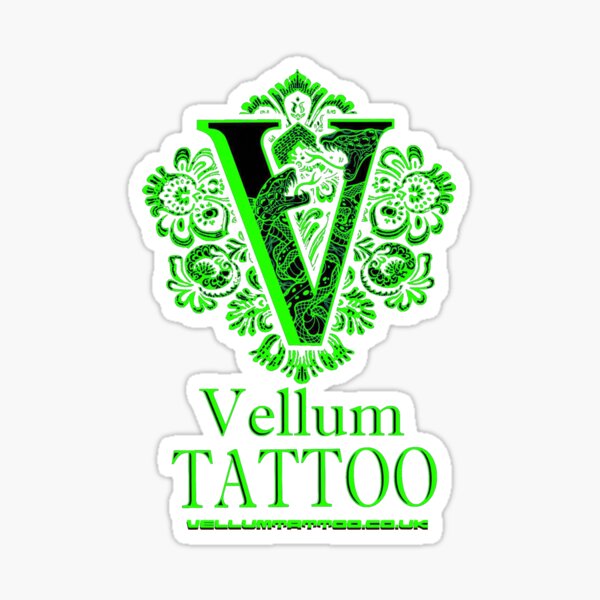The image depicts a sticker or potential patch showcasing the logo for Vellum Tattoo. The centerpiece of the logo is a prominent black letter "V," encircled by intricate tribal floral designs forming a six-pointed flower. Below this central motif, the text "Vellum Tattoo" appears in a bold green font. Further down, the website "vellumtattoo.co.uk" is listed in smaller text. The entire logo is encapsulated within a white outline, giving the appearance of a sticker. The overall color scheme prominently features black and green elements, with a design that conveys both artistic and promotional intent. The jagged edges of the white outline add a cloud-like shape around the sticker, enhancing its distinct appearance. The green tribal floral symbols and the black "V" together create a visually dynamic emblem for the Vellum Tattoo brand.